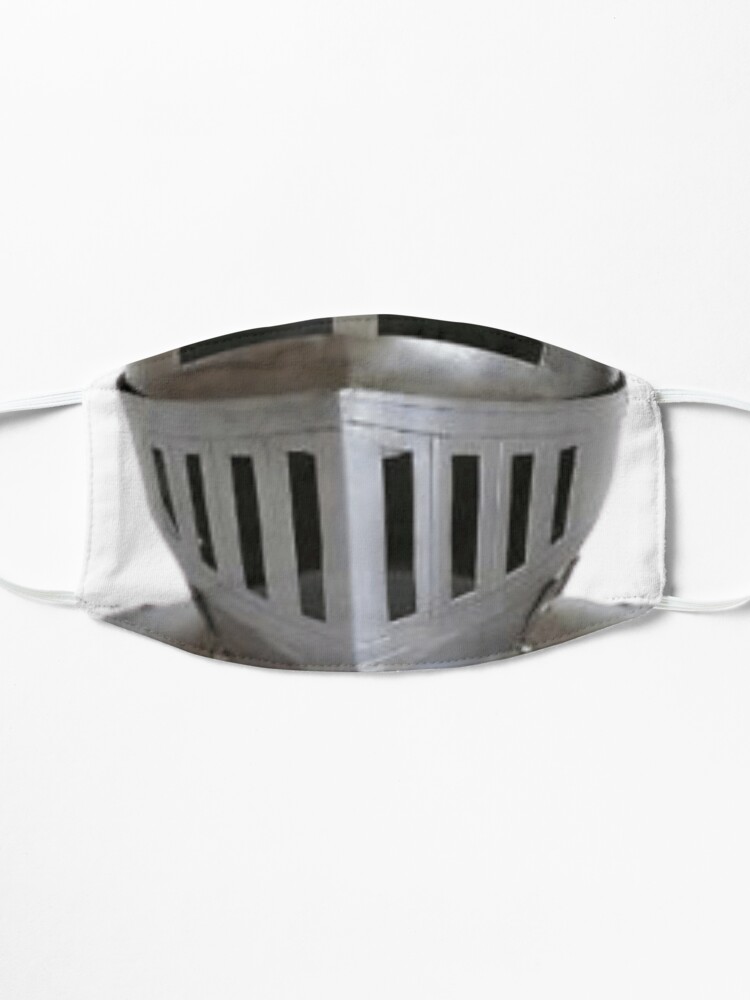The image depicts the bever portion of a medieval knight's helmet, specifically designed to guard the mouth and neck areas. This segment of the helmet features vertical slats that allow the wearer to breathe. The helmet piece, with its dull gray metal and grating that peaks to facilitate both protection and ventilation, occupies a prominent position in the image. Behind this medieval artifact, a modern cloth face mask, with white bands for ear loops and a thicker material suggesting a reusable design, is partially visible. The face mask, likely intended for protection against infectious diseases, is set against a solid white background, contrasting sharply with the grayed metallic armor. The overall image is a vertically long rectangle, roughly two to three times taller than it is wide, presenting a detailed juxtaposition of historical and contemporary protective gear.